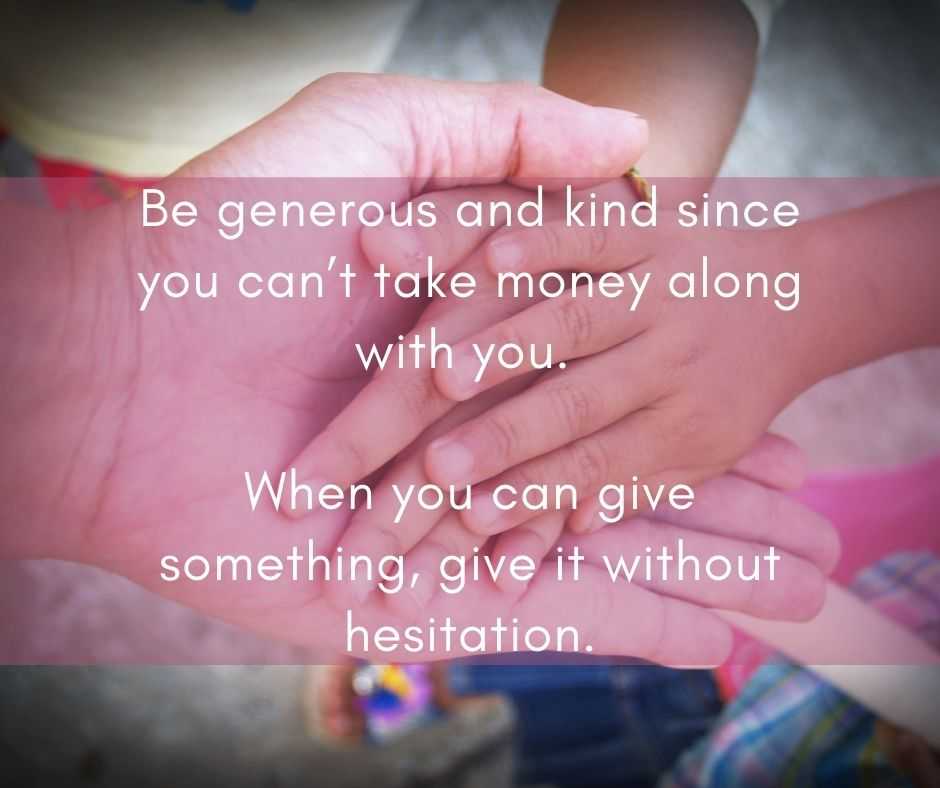The image depicts a poignant scene set against a blurred outdoor background, featuring a close-up of large adult hands with their palms facing upwards, cradling two smaller children's hands. The adult hands appear to be those of a fair-skinned man, while the children's hands exhibit a tanner complexion, indicating diverse ethnic backgrounds. The children's attire is vividly detailed: a boy in a yellow shirt and red shorts, and a little girl in a pink shirt with a blue skirt, complemented by sparkly purple, yellow, blue, and white sandals.

A semi-transparent pink rectangle is centered over the hands, with an inspirational message in white text that reads: "Be generous and kind since you can't take money along with you. When you can give something, give it without hesitation." The intricate details of the children's clothing and the sense of unity portrayed by their joined hands create a heartwarming representation of kindness and generosity.